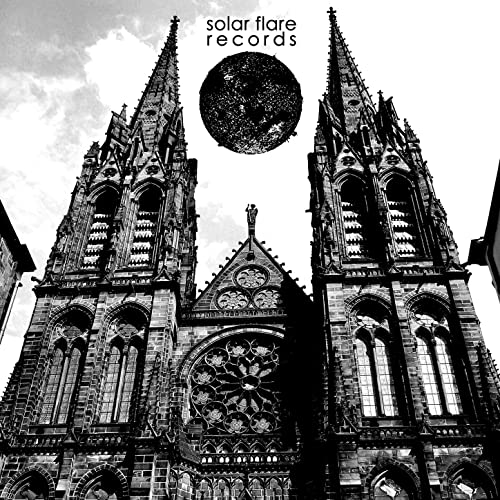The image is a black-and-white photo taken from the ground, angled upwards, capturing a grand, Gothic-style cathedral, reminiscent of Notre Dame. The imposing structure, with its dark stone, features two towering spires adorned with crosses, hexagonal or octagonal in shape, leading to sharp points. The facade is characterized by numerous tall, narrow windows, possibly stained glass, arranged in pairs, with some circular windows interspersed. Between the two spires, the cathedral's central section showcases a large circular window surrounded by smaller circular windows. Above this central section, a moon or planet, adorned with small, white dots, appears to be Photoshopped into a cloudy sky. The top center of the image prominently displays the text "Solar Flare Records" in black. The overall composition is monochromatic, with shades of black, white, and gray, emphasizing the stark, historical beauty of the cathedral against a dramatic sky.